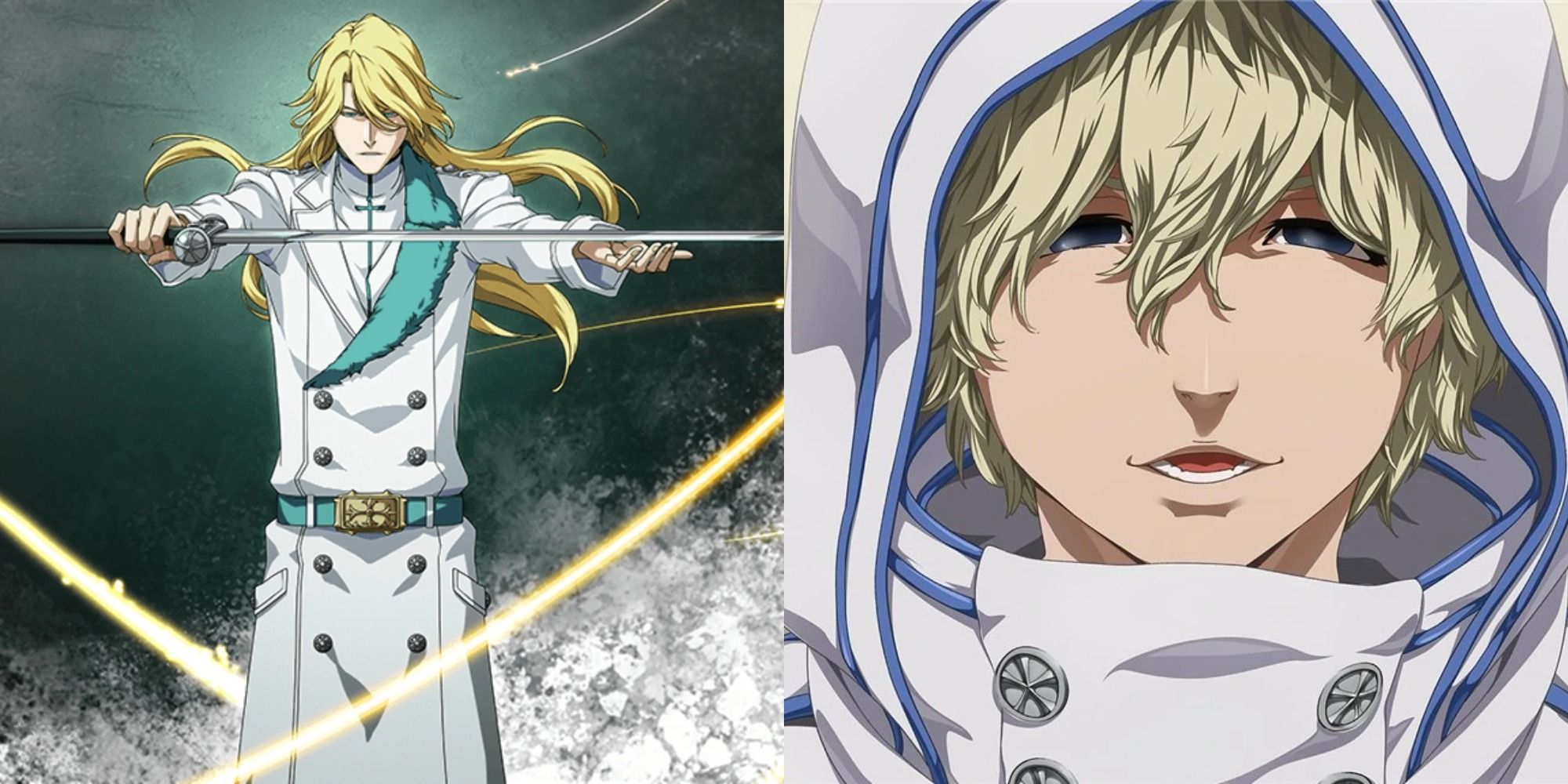This horizontal cartoon image is divided into two panels. The left panel features a full view of a young man with long, flowing blonde hair, standing at the center and facing the viewer. He is clad in a white, double-breasted coat adorned with six to eight goldish buttons, a teal-green lapel on the left side, a green belt with a gold buckle, and possibly a white shirt underneath. He holds a horizontal steel sword with a brown handle, and his hands are positioned with one palm down and the other palm up. Background elements include a radiating green light and dynamic streaks of light surrounding him, suggesting a concentrated, intense moment. The bottom portion of the image appears textured in white and gray tones.

The right panel provides a close-up of what seems to be the same character, now under a white hood trimmed with blue, which reveals a part of his face up to mid-chest. His long blonde hair peeks out beneath the hood, his eyes are dark blue, and his mouth is open, showing his white teeth and reddish tongue. The hooded figure's attire includes two visible buttons and parts of two additional buttons, with the white coat continuing with blue accents. The close-up suggests a different, yet equally focused and intense expression.